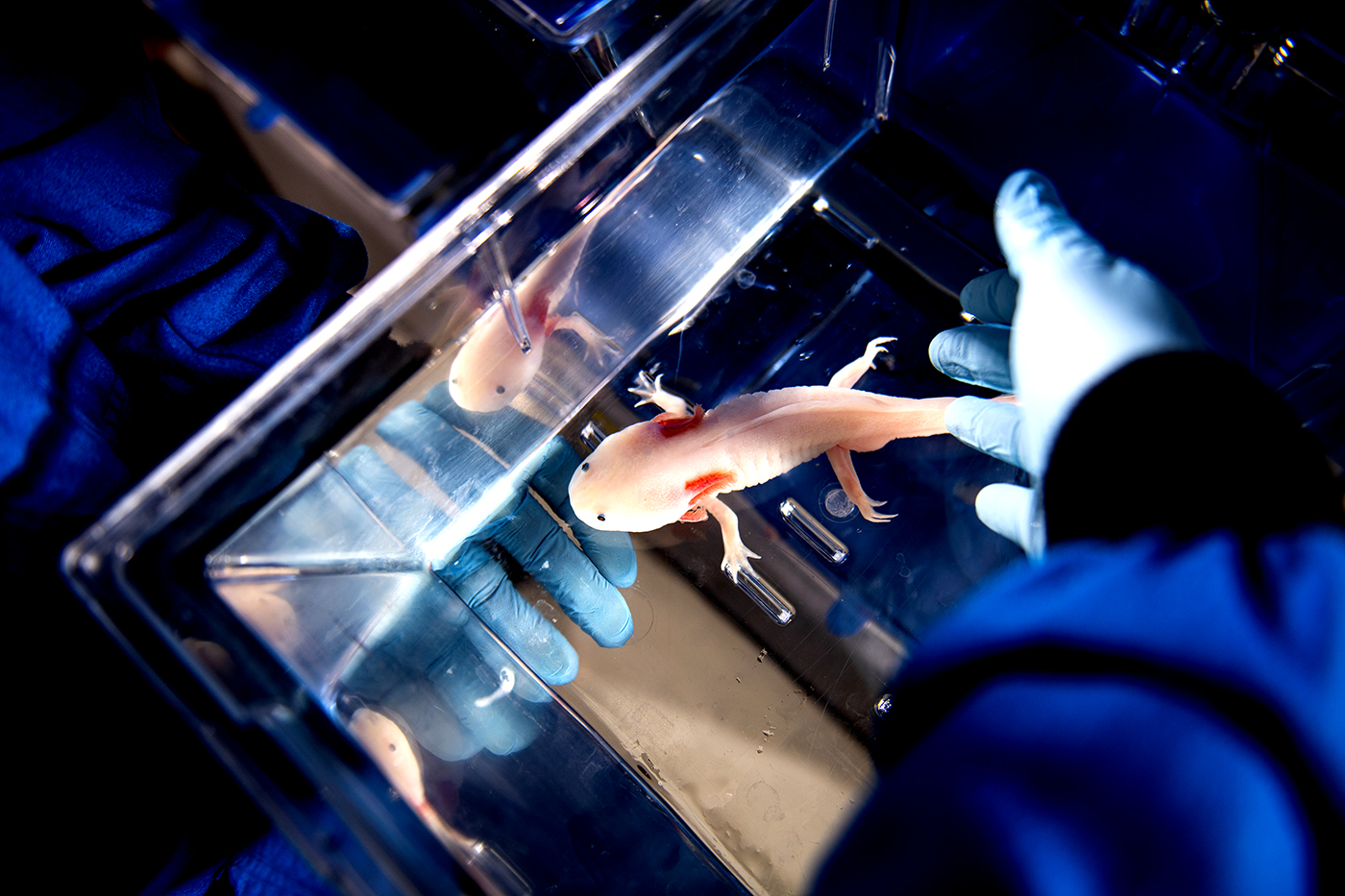In this color photograph, we observe a person, clad in blue long-sleeved attire and green latex gloves, handling a clear aquarium tank. The tank houses a striking peach-colored amphibian, possibly an axolotl, notable for its external gills that resemble red, feathery fins extending from its head. The creature, distinguished by its four limbs and long tail, sits in a tank that seemingly contains water, as indicated by the surrounding environment and positioning of the hands. The individual’s blue-gloved hands are visible both beneath and reaching into the tank, suggesting some interaction or examination. The perspective of the image is downward, showcasing the tank and its inhabitant illuminated clearly under strong lighting, enhancing the detailed view of this intriguing amphibian.